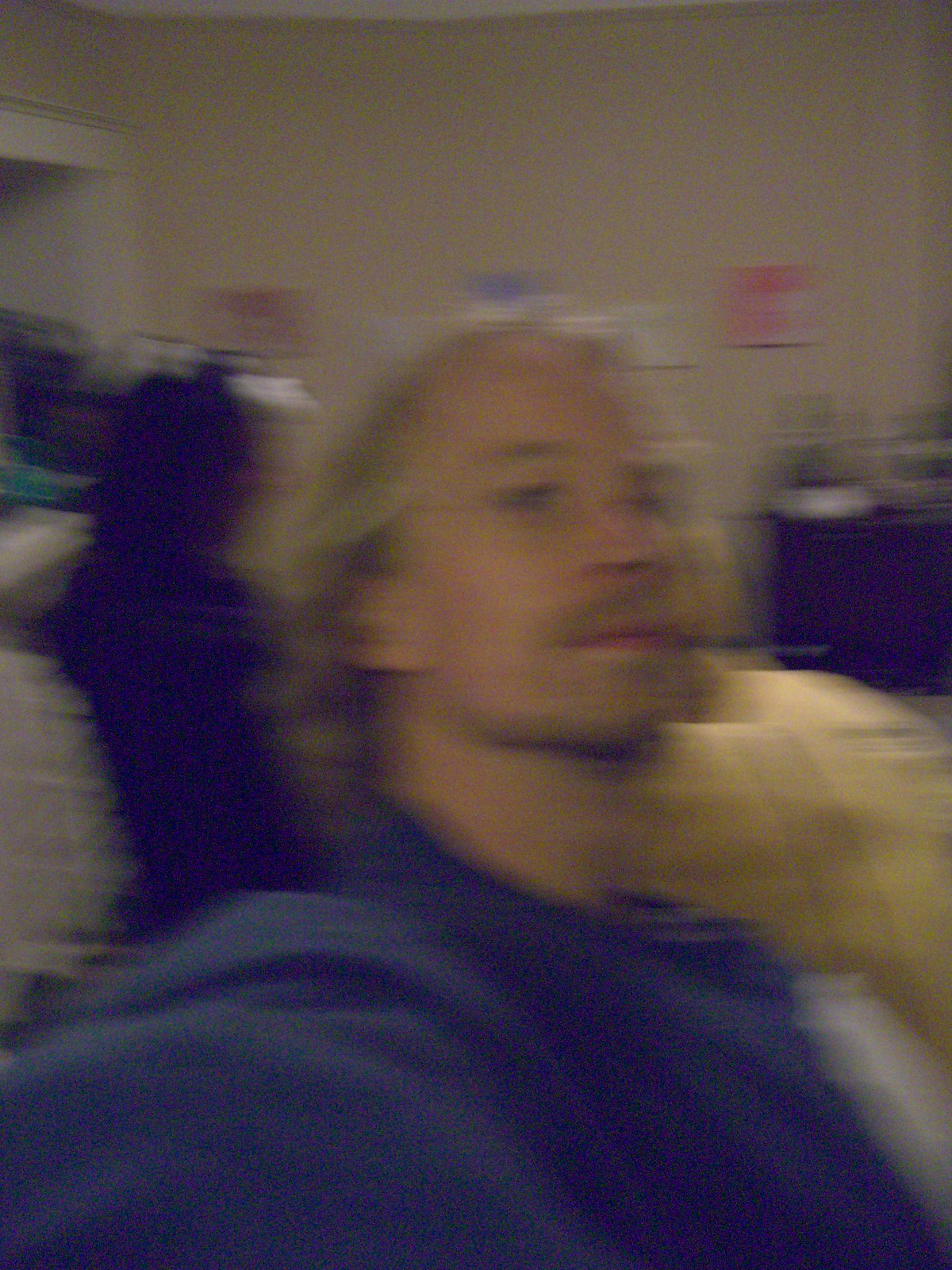This is a blurry photograph of a man with light skin, dirty blonde, shoulder-length hair, and a receding hairline. He has a dirty blonde mustache and a short beard, along with dirty blonde eyebrows. He appears to be holding the camera in his left hand and is wearing a dark blue long-sleeved sweatshirt. The man is sitting on a tan couch that is very blurred, making it difficult to discern with certainty. Behind him, there are various indistinct items including black clothing, some boxes, and a plant on a dark chocolate brown or black desk. The blurred background also features paintings in white, pink, and hot pink colors, as well as a black dog, and an open door frame lined with white wood. The walls are cream-colored. The overall quality of the image is poor, making specific details challenging to identify.